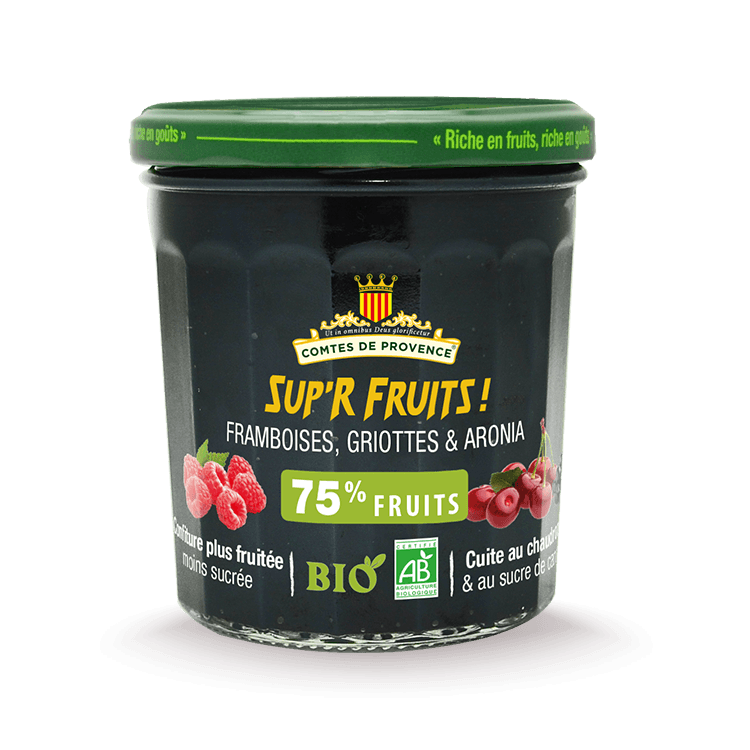The image depicts a jar of French jam or jelly from "Comte de Provence" with a detailed and vibrant design. The jar itself is dark, almost black in color, and is not see-through, suggesting its dark red or blue content. The lid is green, adorned with French text that reads "riche en fruits." At the top of the jar, there is a crest featuring a crown and yellow and red stripes, surrounded by golden scrollwork. Below the crest, "Sup'R Fruits!" is prominently displayed in yellow letters, followed by the fruit varieties "framboise," "griottes," and "aronia." A green banner in the middle of the jar declares "75% Fruits" in white capital letters. The left side of the jar shows an image of red raspberries with green leaves, while the right side features six cherries with stems and a single green leaf. Below these images, the word "bio" is written in green with leaves accenting the letter "O." Additional French text and a white "AB" logo are also visible, emphasizing the organic nature of the product.